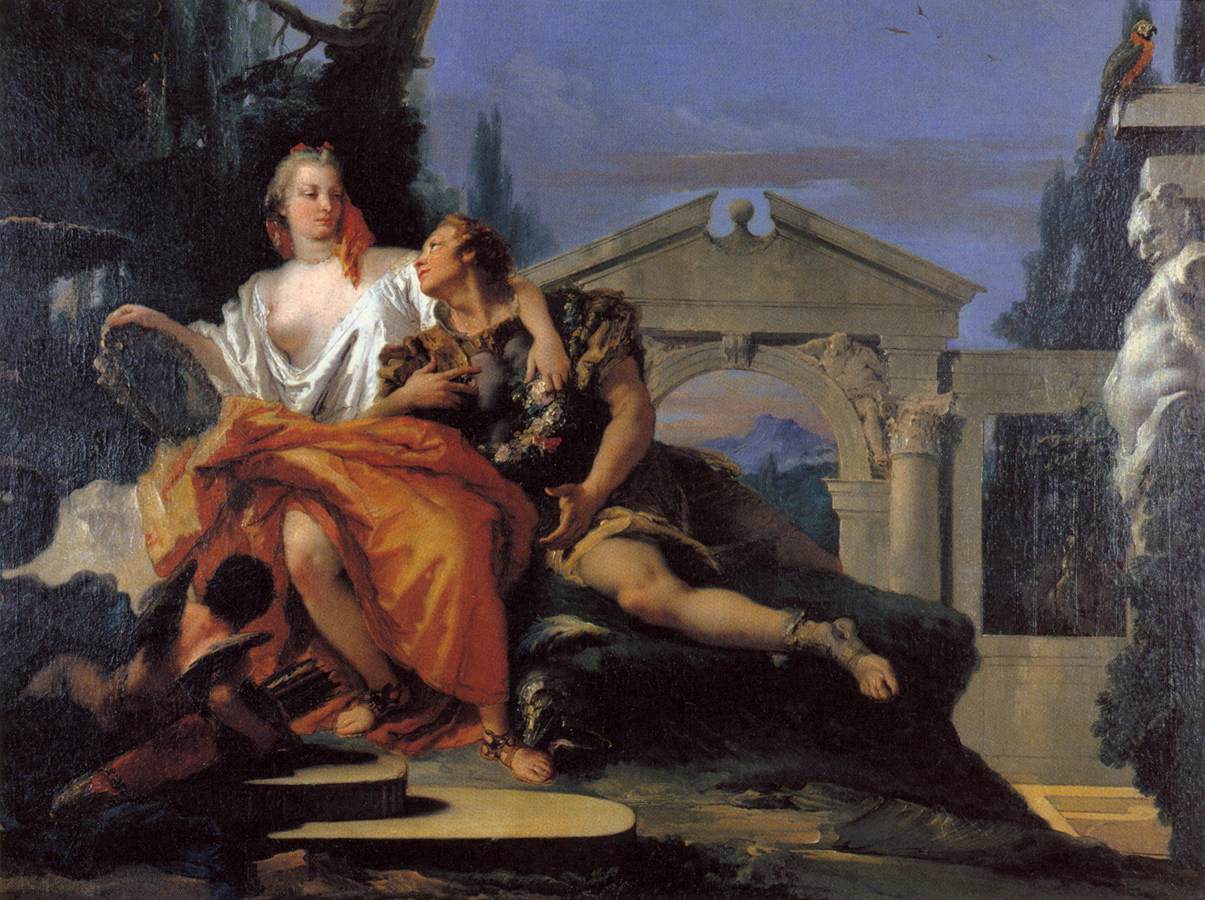The painting, reminiscent of Renaissance art, features a romantic scene between a woman and a man seated on a rocky outcrop. The woman, positioned on the left, is elegantly clothed in a white blouse and an orange full skirt, her right knee and feet exposed, adorned with footwear. A red ribbon or headscarf adorns her tied-up hair, contrasting with her exposed right breast. Cradled in the woman's arms, the man, dressed in gray and brown warrior attire with visible right leg, gazes up at her while seemingly engaged in conversation. 

The woman's left hand tenderly holds a circular object, possibly a mirror or shield, and at her feet lies a small winged devil-like figure, resembling a cherubic Cupid, clutching a quiver of arrows. Near this cherub, the man's helmet is also visible. A temple-like gateway, cream-colored with an arched doorway, dominates the background, flanked by trees and bushes. On the right side, a white statue capped by a pillar with a perched parrot, adds an element of classical antiquity. Above, the sky, painted in shades of dark blue and streaked with clouds, suggests the fleeting moments of dawn or dusk, with birds flying in the distance, enhancing the painting's ethereal and timeless quality.